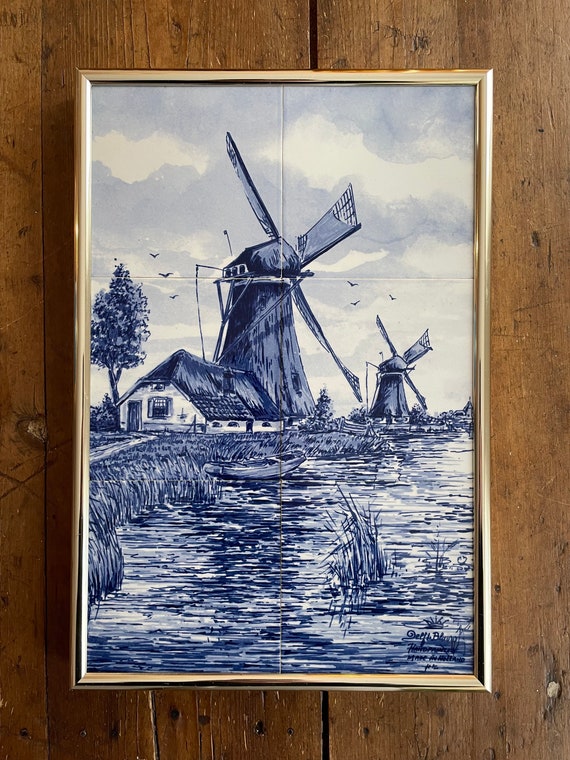The image is of a detailed blue and white painting on six framed tiles, two wide by three tall, resting on a weathered wooden table with a walnut stain, characterized by its shiny, medium brown color and distressed, darker tones. The painting, enclosed in a gold frame, depicts a serene scene with a large central windmill and a smaller windmill to the right. Beneath the larger windmill sits a small house, possibly a barn or a Dutch yurt, with a tree beside it. The house features a front door, a window, and a side window. Birds can be seen flying in the blue and white watercolor sky. In front of the house, there are reeds, grass, and a walkway leading to a waterway that flows from the left to the right, with a small rowboat and emerging weeds in the water. The signature on the bottom right corner of the artwork is illegible.